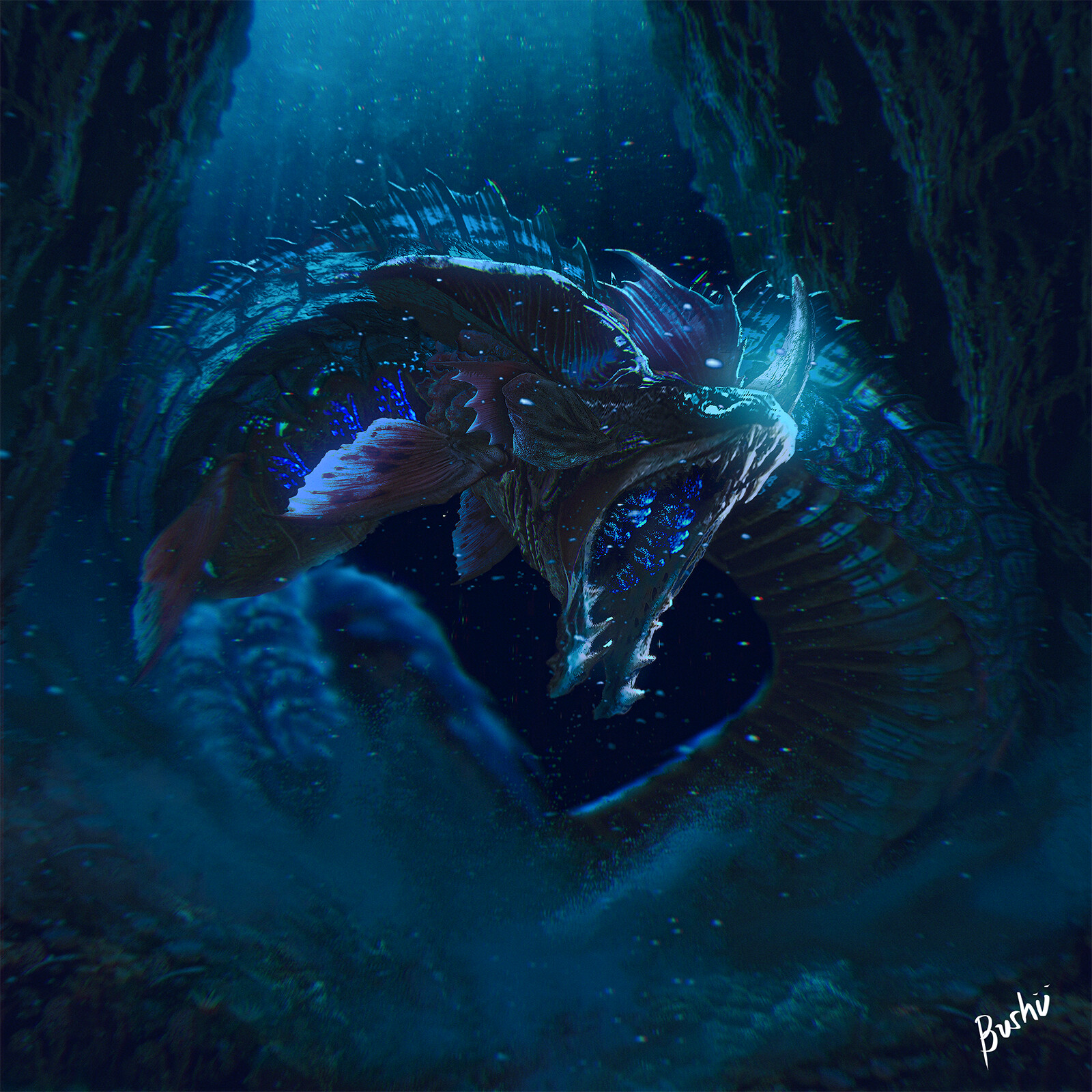The image depicts a scene resembling a digital painting set in an underwater cave. At the center is a formidable, snake-like sea creature with a long, coiled body that swirls around, stirring up a dust cloud along the cave floor. The creature's head features a prominent, bioluminescent horn glowing with a whitish-cyan light, positioned at the top center of its nose. Fins akin to those of a fish protrude around its gills, just above the head, adding to its monstrous appearance.

The creature's mouth is agape, revealing an array of massive teeth along both the upper and lower jaws, suggesting it is actively hunting or warding off intruders. The interior of its mouth glows with a dark blue hue that continues along the bottom of its head. The creature's slitted eyes complete its intimidating visage. 

The surroundings emphasize the sea creature's domain, with rock formations framing the scene on either side, reinforcing the notion that this menacing inhabitant is guarding its underwater territory.